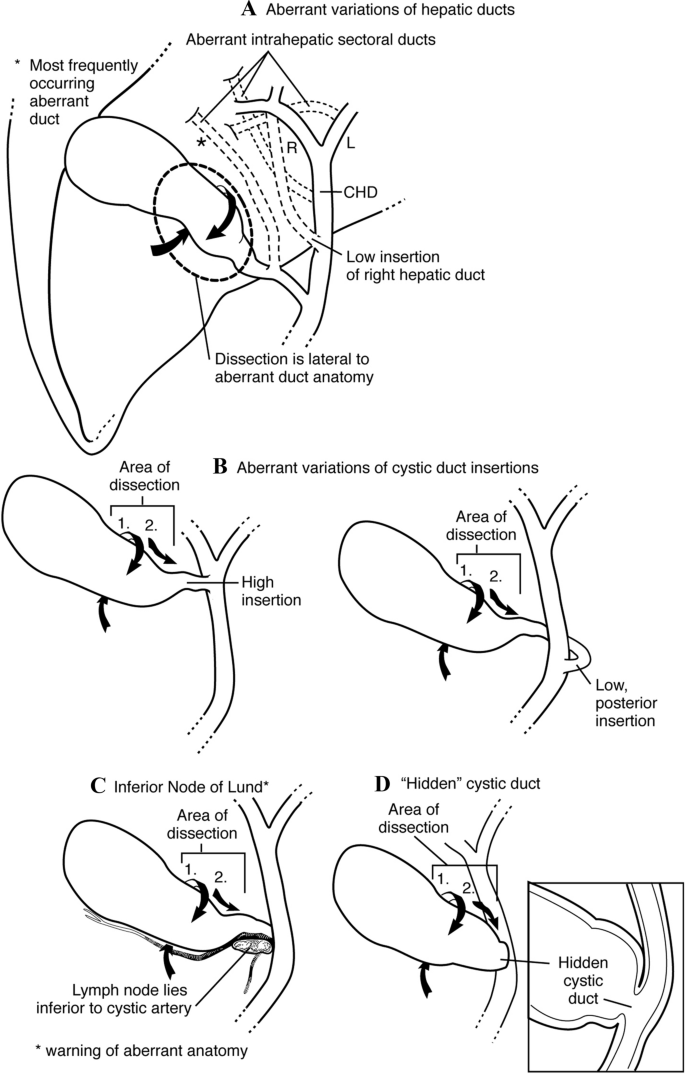This is a detailed black-and-white medical illustration, designed to instruct surgeons in addressing a condition involving aberrant duct anatomy. The diagram, which appears to come from a medical textbook, is laid out on a white background in portrait format, with the dimensions making the top and bottom shorter than the sides. The illustration includes several labeled sections: A, B, C, and D, each accompanied by smaller diagrams and descriptive text.

At the top, bold black text reads "Aberrant Variations of Hepatic Ducts" and "Aberrant Intrahepatic Sectoral Ducts". Section A highlights "most frequently occurring aberrant duct" and denotes "Low insertion of right hepatic duct dissection is lateral to aberrant duct anatomy." This section seems to feature depictions of veins and ducts with detailed annotations.

Section B discusses "aberrant variations of cystic duct insertions," illustrating different types such as high insertion and low posterior insertion, with areas of dissection indicated by dashed lines and arrows.

Section C, located in the lower left-hand corner, identifies the "Inferior Node of Lund" and includes notes about dissection areas and the lymph node's position relative to the cystic artery.

Section D on the right focuses on the "hidden cystic duct," providing a zoomed-in view within a square box to give additional details on this component.

Overall, the diagram is clearly focused on providing surgical guidance for handling ducts that are aberrantly positioned or otherwise problematic, emphasizing the need for dissection to resolve blockages and fluid buildup. The various detailed annotations and supplemental diagrams serve as a critical reference for surgeons aiming to navigate this complex anatomical terrain.